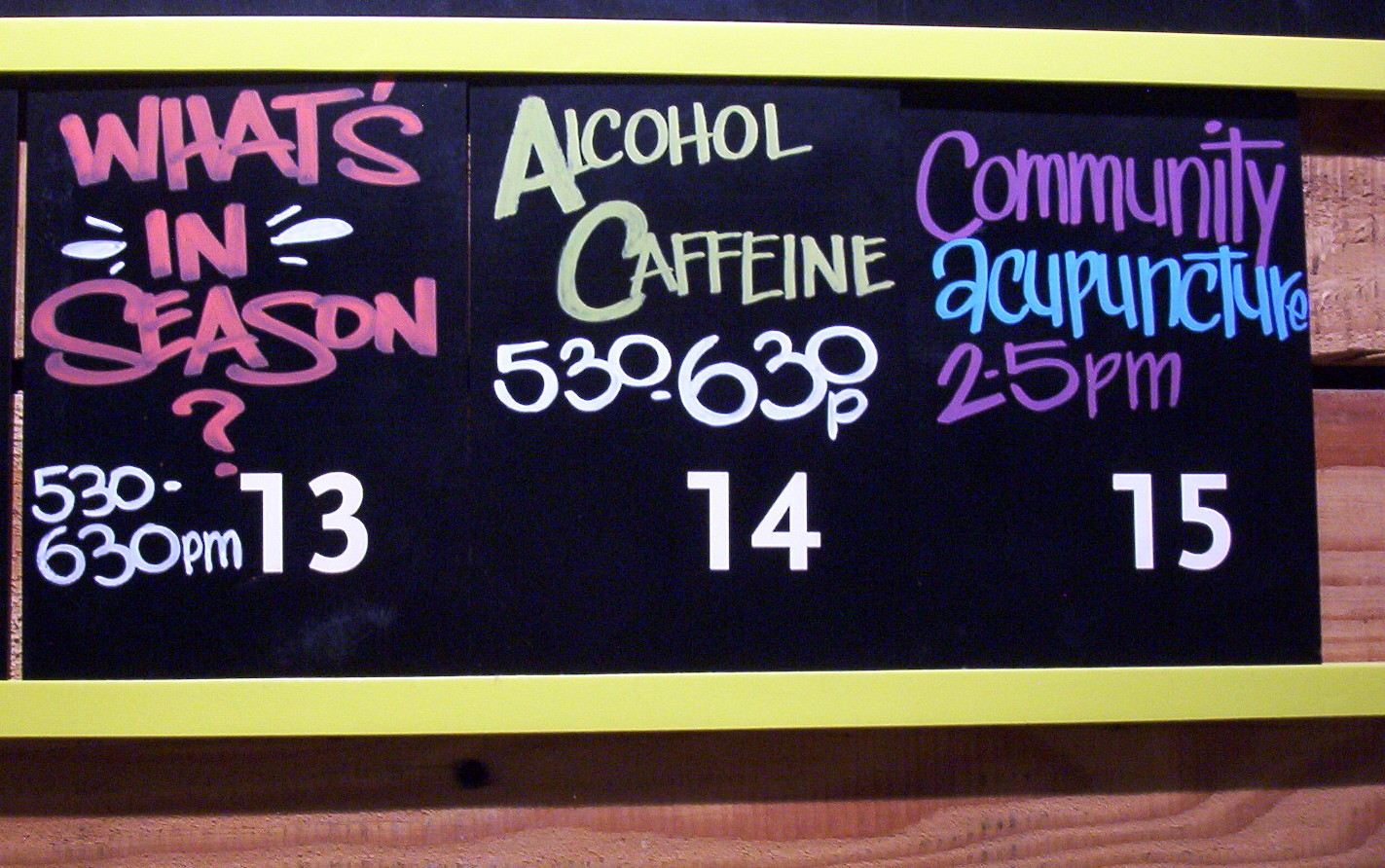The image features a close-up view of a sign displayed on a wood-slatted wall, framed by a yellow beveled border. The sign is divided into three closely placed black blocks, each with colorful text indicating different events and times. The first block, adorned with large capital pink letters and decorative white dashes, reads "WHAT'S IN SEASON" followed by the time "5:30 to 6:30 PM" and the date "13" in large white block numbers. The center block features light yellow letters stating "ALCOHOL, CAFFEINE," with the time "5:30 to 6:30 PM" and the date "14" in large white block numbers. The third block displays the word "COMMUNITY" in purple letters, followed by "ACUPUNCTURE" in light blue, with the time "2 to 5 PM" and the date "15" in large white block numbers. This colorful and detailed sign provides a clear schedule of various activities.